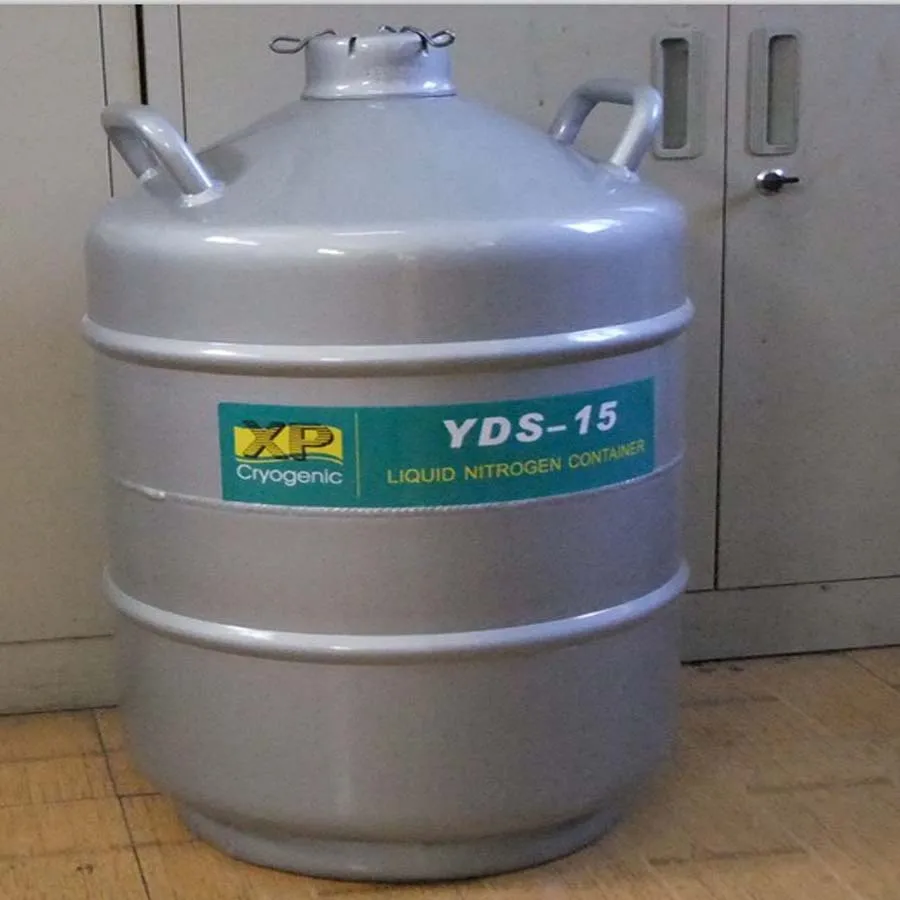The square indoor photograph prominently features a shiny, gray, tub-like container resembling a small propane tank, approximately 5 gallons in size, resting on a honey-colored parquet floor. This tank has two large handles on either side of its upper section and a lid secured with clips. The middle of the tank displays a green label with the text “YDS-15” in white, “liquid nitrogen container” in yellow beneath it, and to the left, the letters "XP" with the word "cryogenic" below. In the background are gray, smudged locker-style cabinets with matching gray handles and a visible lock mechanism near the bottom.